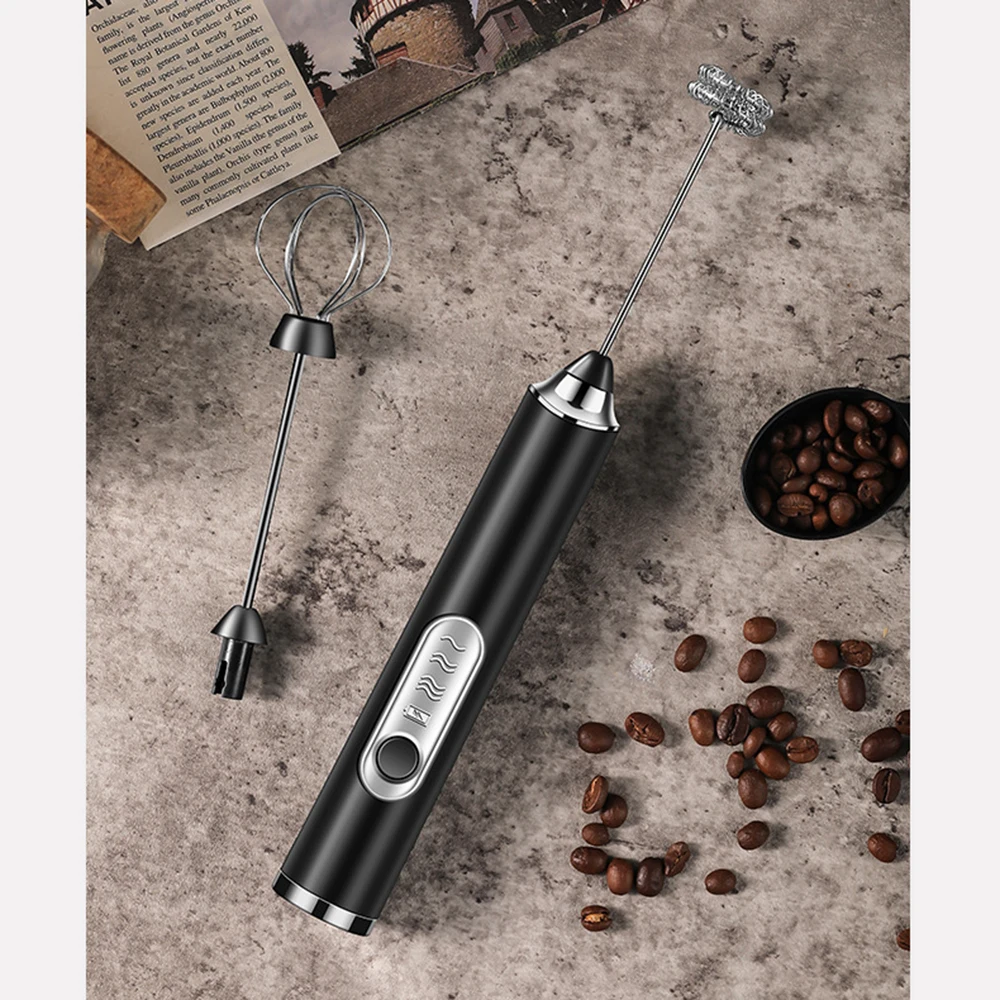This top-down photograph showcases a black and chrome handheld milk frother prominently displayed on a marble countertop, suggesting a product advertisement. The frother features a single black circular button and visible four settings, indicative of its automatic functionality. Positioned beside the frother is an alternate attachment resembling a small whisk, while the main attachment consists of two spiraled, curled discs like a spring. Surrounding the frother, a black spoon filled with coffee beans and loose beans scattered across the countertop emphasize a coffee-making theme. Additionally, the top left corner subtly reveals a book with imagery potentially depicting an ancient Roman or European castle, adding a touch of sophistication to the scene.